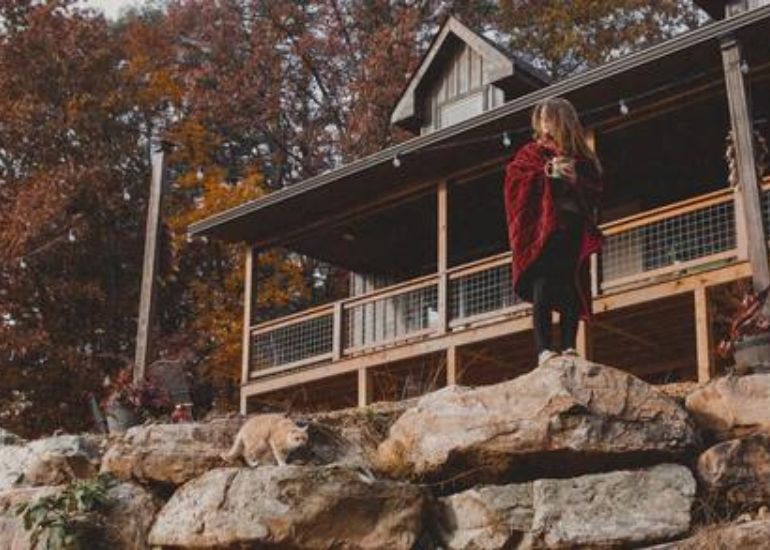In this grainy, autumnal photo, a young woman with long, light brown hair stands on a rocky ledge in front of a tranquil wooden cabin. She is dressed in a red shawl draped over her shoulders and black leggings, holding a coffee mug and gazing into the distance. The scene is set against a backdrop of tall trees shedding their red, brown, and yellow leaves, indicating the season is fall. Beside her on another rocky outcrop sits an orange cat with white fur on its chin and paws. The cabin behind her appears to be dark brown, one-story with an attic, and it features a large front porch. The atmosphere suggests a serene and cool fall day, with the woman seemingly enjoying the tranquil, forested surroundings.